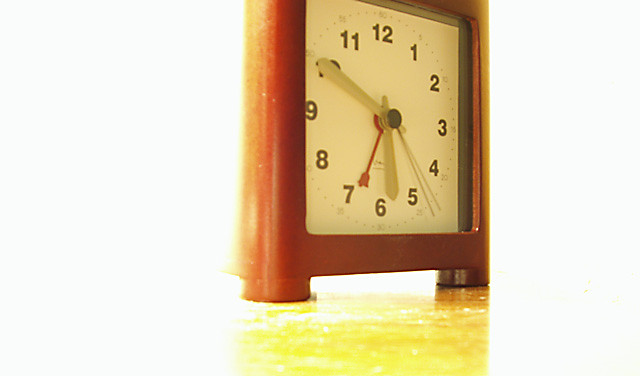This photograph captures a classic desk clock with a white clock face. The clock features bold black numerals marking each hour from 12 to 11, arranged in a circular pattern around the face. Interspersed between these hour markers are smaller, lighter grey numerals that indicate the seconds, starting with 60 above the 12, then proceeding in increments of 5 (5, 10, 15, etc.) around the dial. The brand name, situated above the 6, is indistinct and difficult to decipher due to the photo's slight blur, suggesting it might be an older image. The clock's wooden frame adds a touch of warmth and elegance, complemented by its small, rounded feet that keep it securely perched on the desk. The desk itself appears to be made of a light-colored wood, harmonizing perfectly with the clock's vintage aesthetic.